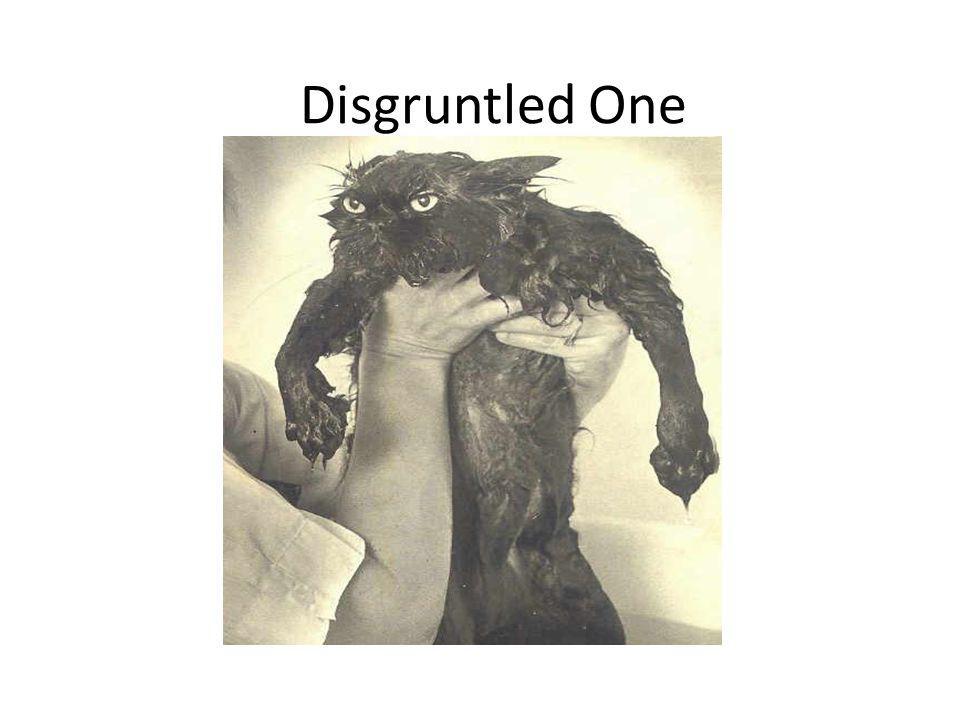The image is a black and white, vintage-style photo, measuring four inches by four inches, with a grainy, lower quality. It features a wet, black cat being held up by a person's arm, wrapped in a white short-sleeved shirt. The photograph captures the feline's extremely angry and disgruntled expression, with its ears pointed to the side and its body dripping wet, likely from a recent bath. The cat's front paws are splayed out to either side, giving it an almost bodybuilder-like stance. Above the cat, in bold black lettering, reads "Disgruntled One." A slight vignette effect edges the photo, enhancing its old-fashioned appeal. This humor-infused image, reminiscent of popular Facebook or Instagram posts, can serve as a light-hearted, non-offensive icebreaker in professional or casual settings, playing on the universal charm of grumpy cat photos.